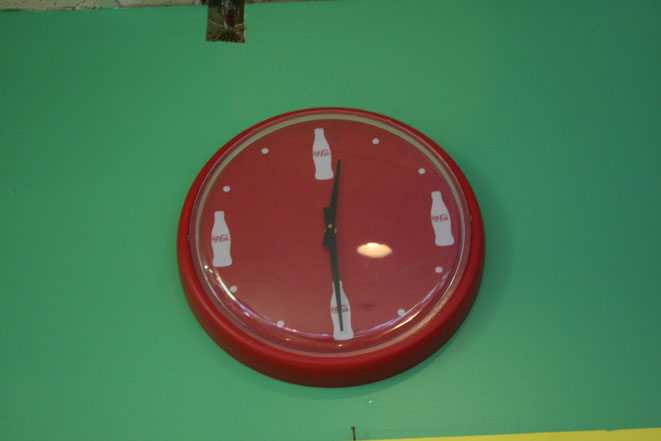The image showcases a vintage Coca-Cola wall clock prominently displayed on a green wall, tinged with subtle hints of yellow at the bottom, partially obscured. The clock is distinctively round with a vibrant red face, and it features classic Coca-Cola branding. At the top of the clock, marking 12 o’clock, is a miniature 3D Coca-Cola bottle. The clock’s hours are represented at 3, 6, and 9 o’clock by similar Coke bottles, while smaller dots indicate the hours in between. Unlike traditional clocks with numerical markers, this nostalgic design exclusively uses Coke bottles and dots to denote the time. The clock face is encased in a clear plastic cover, indicative of its antique status. The clock hands, simple and black, point in their respective directions to display the current time.